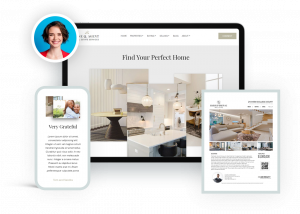This screenshot showcases a real estate website displayed across various devices and formats, highlighting its responsive design. 

At the top left, there is a circular profile picture of a woman with short brown hair, set against a blue background and encircled by a white border. To the right of this profile picture, a monitor mock-up displays the website's interface. The website features a white navigation bar at the top, with the company logo positioned on the left side. There are six clickable links in the navigation bar, with an additional possible link situated on the far right.

Beneath the navigation bar, a banner reads "Find Your Perfect Home," accompanied by a series of interior photographs showcasing various home styles. 

In the bottom left corner of the screenshot, a phone mock-up presents a partial view of the website, signifying its mobile-friendly capabilities. To the bottom right, another image displays the website interface from a different perspective.

The overall layout underscores the versatility and accessibility of the real estate website across multiple devices.